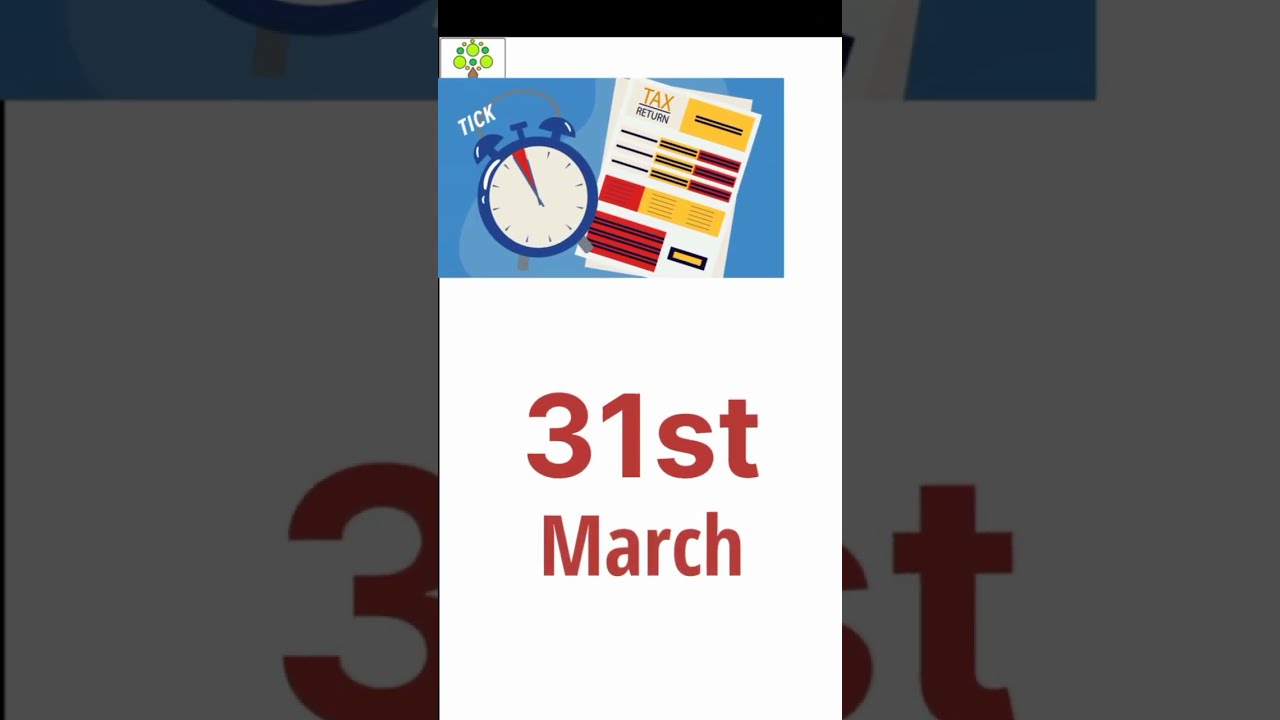The image is a vertical rectangular slide or poster with a predominantly white background. At the top, there is a small blue rectangle featuring an old-fashioned, wind-up alarm clock turned sideways, with a little red mark near the 12 o'clock position, suggesting it's almost midnight. Above the clock, in white italicized uppercase letters, it reads "TICK." To the right of the clock, within the blue rectangle, are images of several tax return forms adorned with various colored blocks—yellow, red, and orange—each with dark borders. Below this blue section, "31st March" is prominently displayed in a maroon or reddish-brown font, indicating a significant date. The overall style suggests that it is an advertisement or reminder for tax season, with the central elements—the clock, tax documents, and date—designed to stand out against the subtle, shaded backdrop.